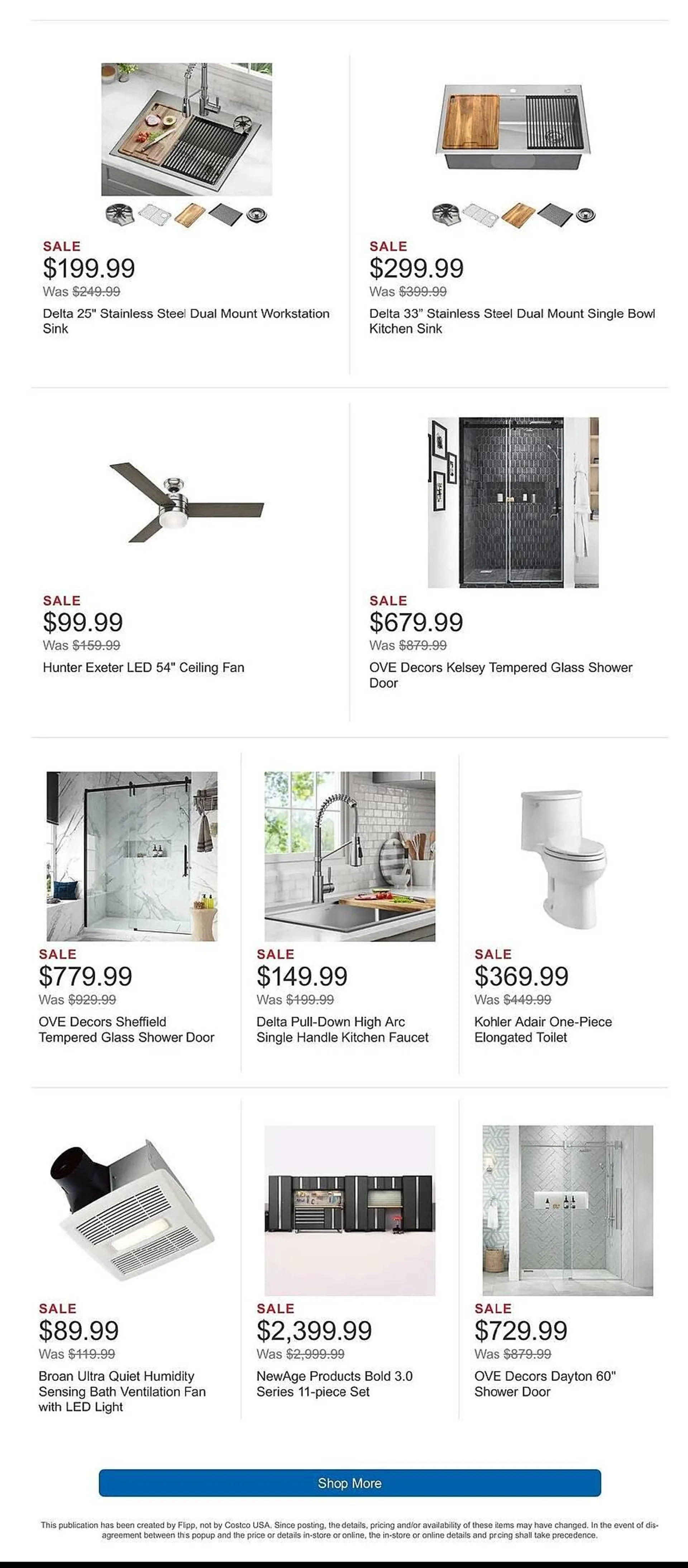A detailed caption for the image could be:

"This image displays a webpage viewed on a mobile device, showcasing various home improvement items available for sale at a home improvement store. The top section features images of sinks, followed by a toilet, shower enclosure, and shower doors. Each item includes a brief description and the sale price prominently displayed. Depending on the image size, the layout presents either two or three items per row. 'SALE' is highlighted in bright red, ensuring it catches the viewer's attention. At the bottom, a blue strip reads 'Shop More,' leading to additional products. Below this, in fine print, there is a disclaimer noting that the publication is created by 'Flip or Fip' and not by Costco, indicating that the items may be sourced from Costco.”